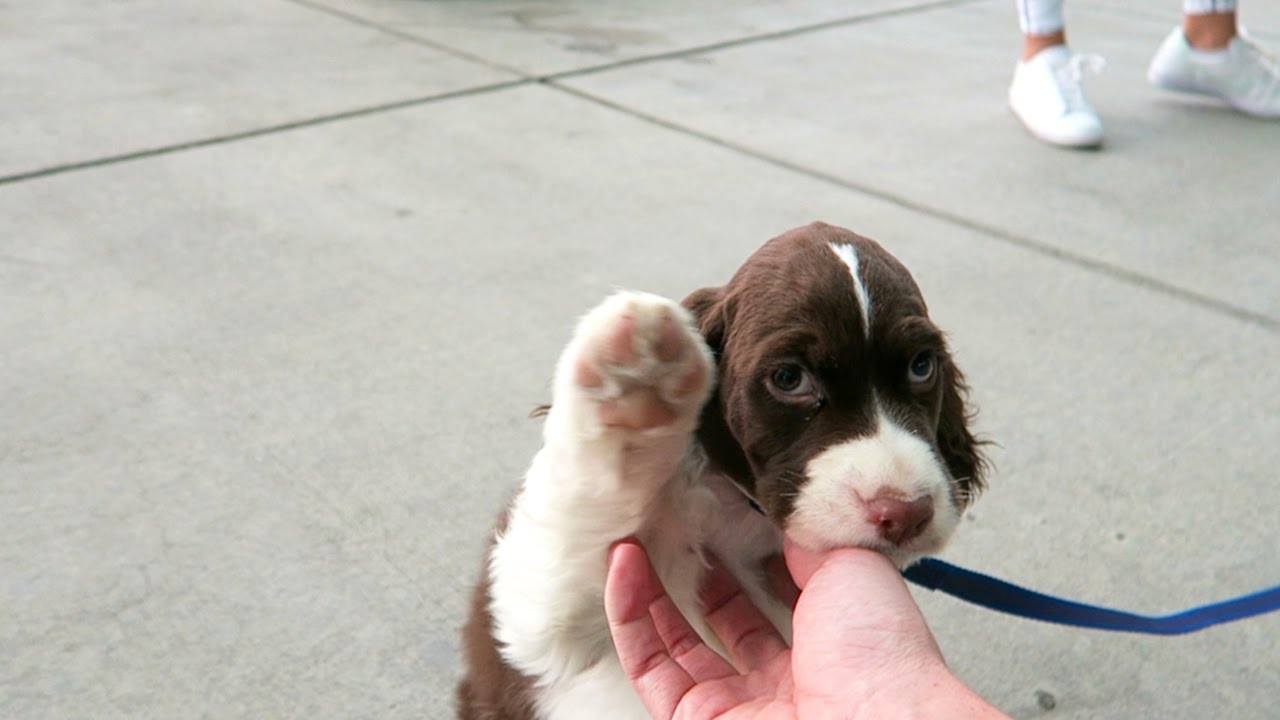In this captivating photograph, a young puppy, likely a Cocker Spaniel or Springer Spaniel and approximately two months old, stands on a city sidewalk. The adorable pup features a mix of brown and white fur: its head and ears are predominantly dark brown, with a distinctive small white strip running between its eyes and halfway up its forehead. The puppy's muzzle is half brown with a white nose, and its pink nose adds a charming detail. Additionally, it sports a white chest and legs. One of its front paws is endearingly raised, creating the impression of a friendly wave towards the camera.

The puppy is secured with a blue leash that trails off to the right side of the photograph, leading out of the frame, leaving the leash holder unseen. Simultaneously, a right hand, presumably belonging to a passerby, is seen scratching the puppy underneath its chin and chest, much to the pup's evident delight.

In the upper right corner of the image, the legs of a person wearing white sneakers and tight blue jeans are visible, suggesting the urban setting of the scene. The clean sidewalk further emphasizes the focus on the sweet interaction between the puppy and the person. This detailed portrayal captures a heartwarming moment of affection on a bustling city street.